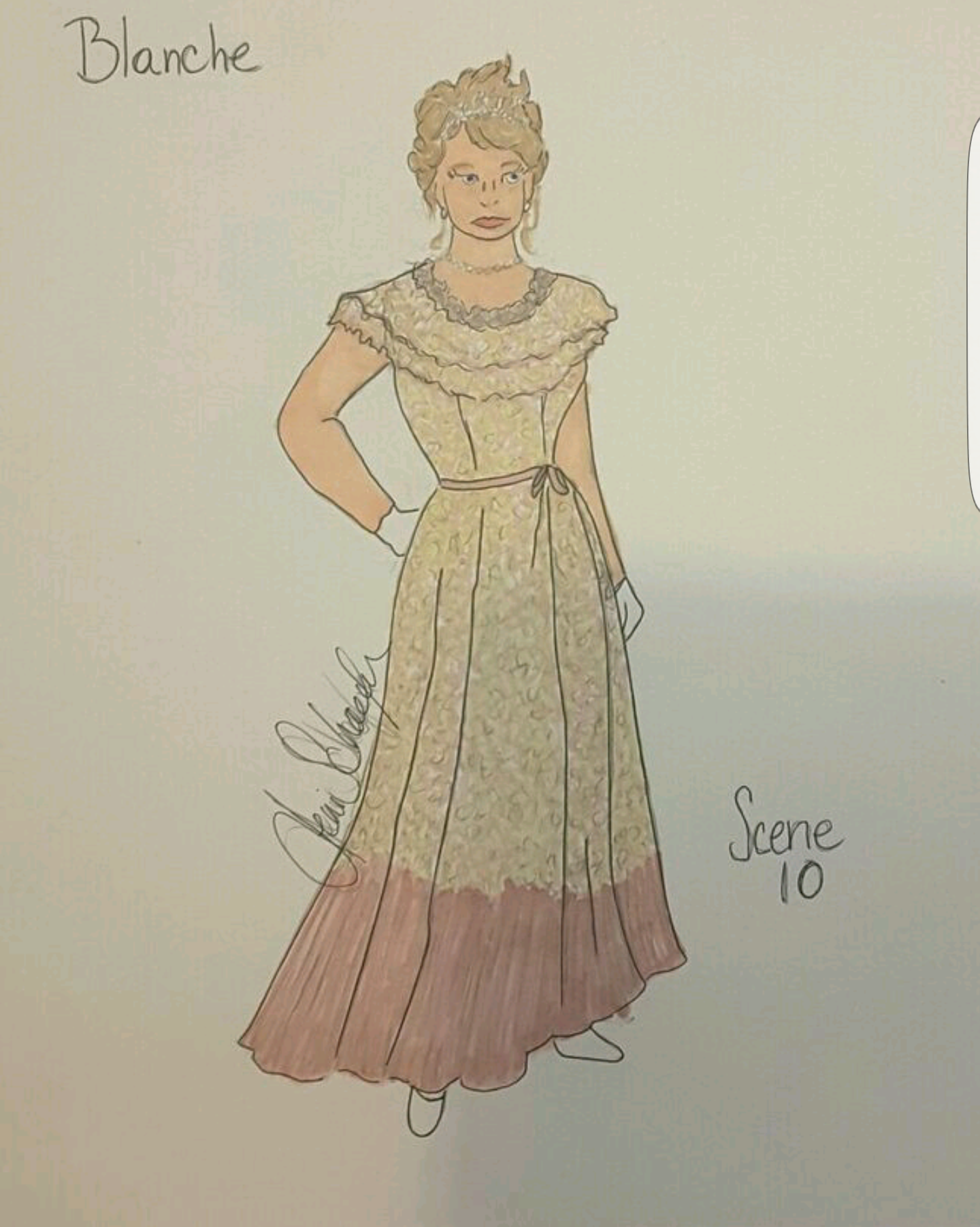The image is a detailed sketch on paper of an elegantly dressed woman named Blanche, as indicated by the handwritten name in the top left corner. The bottom right corner reads "Scene 10" and features the artist's signature, Jen Schaefer. The woman has blonde hair pulled back, adorned with a tiara, and she is depicted with a melancholic or slightly annoyed expression. She is wearing a golden dress with a pinkish bottom, characterized by its ruffled top, short frilled sleeves, and laced with a pink bow at the waist. Her accessories include a diamond necklace, dangling gold earrings, and white gloves. She completes her look with white shoes. The background is a subtle off-white, highlighting the detailed, elegant costume design likely meant for theatrical use.